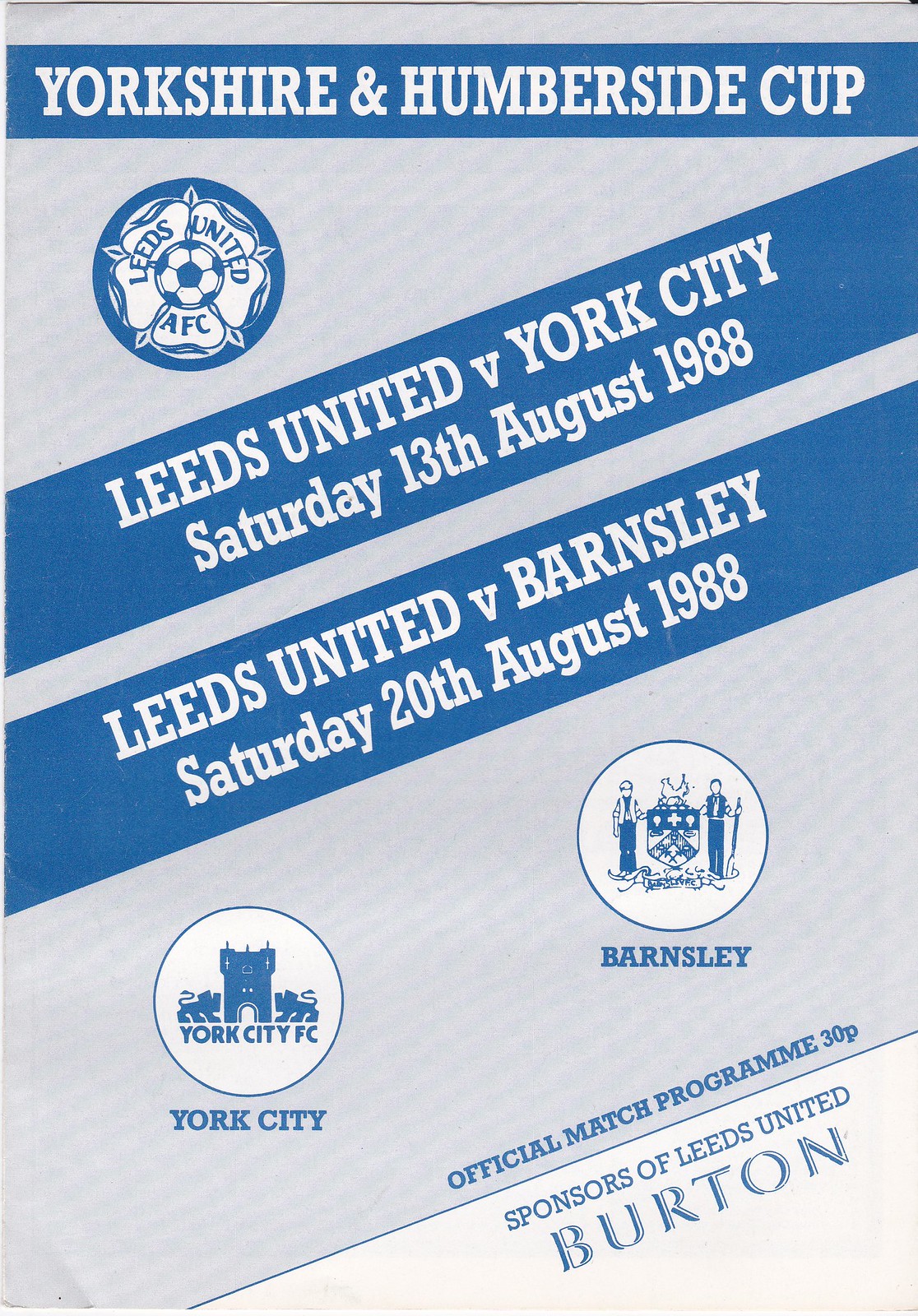The image is a faded, light blue official match program for Leeds United AFC featuring the Yorkshire and Humberside Cup. The program, primarily in blue and white with a pinkish hue, displays a round soccer emblem at the top. Below, it announces two matches: Leeds United versus York City on Saturday, August 13, 1988, and Leeds United versus Barnsley on Saturday, August 20, 1988. Each match is listed within blue bands angled upward to the right. The bottom section of the program contains insignias for York City and Barnsley, alongside "Official Match Program" in blue writing. The sponsor, Burton, is prominently featured in larger blue text toward the bottom. The overall design has a distinct 1980s aesthetic, characterized by its faded colors and angular layout.